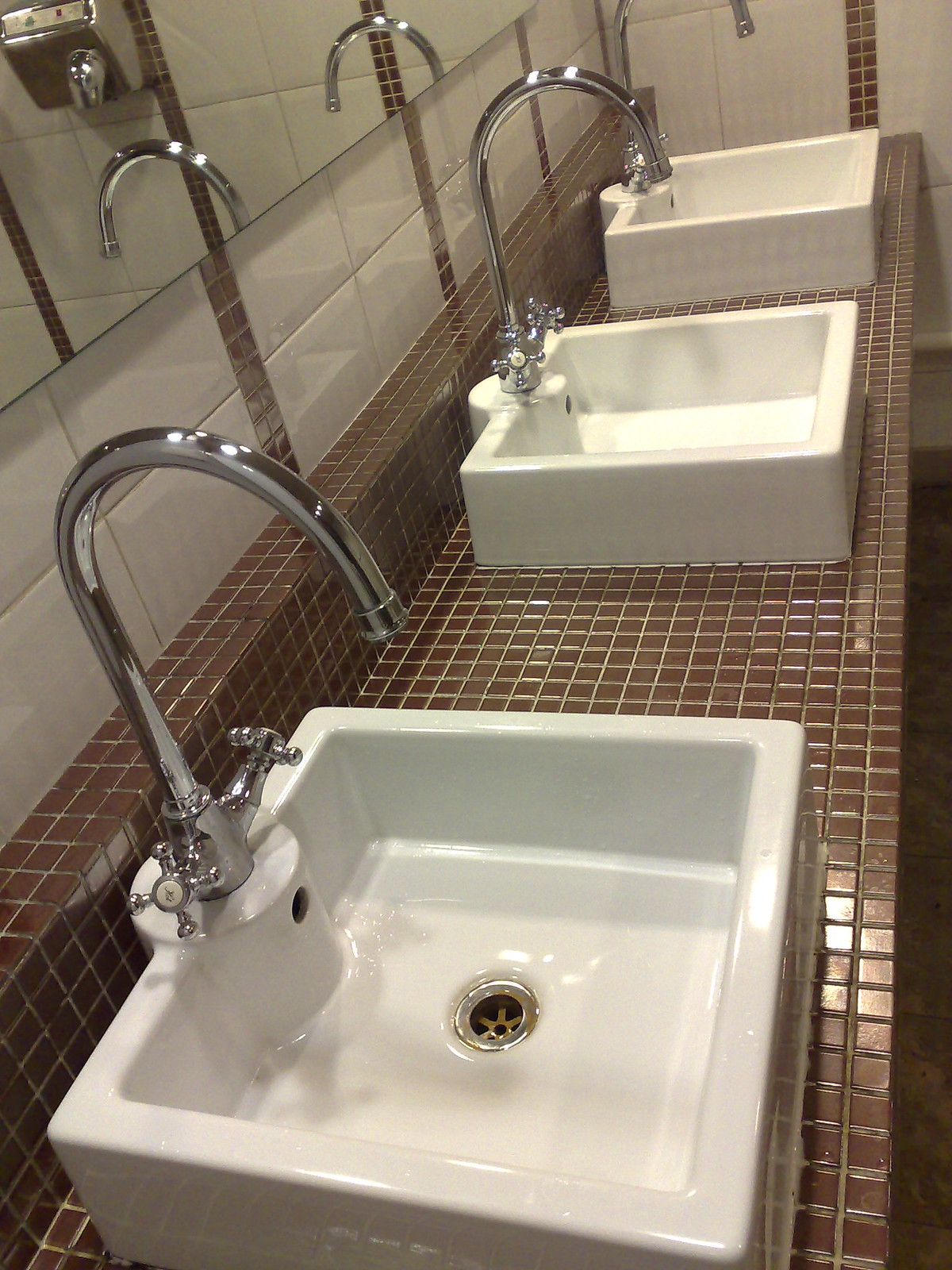The photograph captures the sink area of a commercial public restroom, likely in a restaurant or similar establishment. The image, vertically rectangular, prominently features a countertop made of small square brown tiles, with three white, square porcelain sinks mounted on top. Each sink is equipped with a large gooseneck silver faucet and separate round handles for hot and cold water. The countertop narrows towards the top of the frame, creating a perspective where the front sink is closest to the viewer.

Above the sinks, the wall is adorned with larger off-white or beige tiles accented by smaller brown tiles, which match the countertop's tiles. A mirror is mounted in the upper left corner stretching above the sinks, reflecting the image of a silver hand dryer mounted on the opposite wall. This detailed arrangement of sinks, tiles, and fixtures confirms the setting as a well-maintained commercial bathroom.